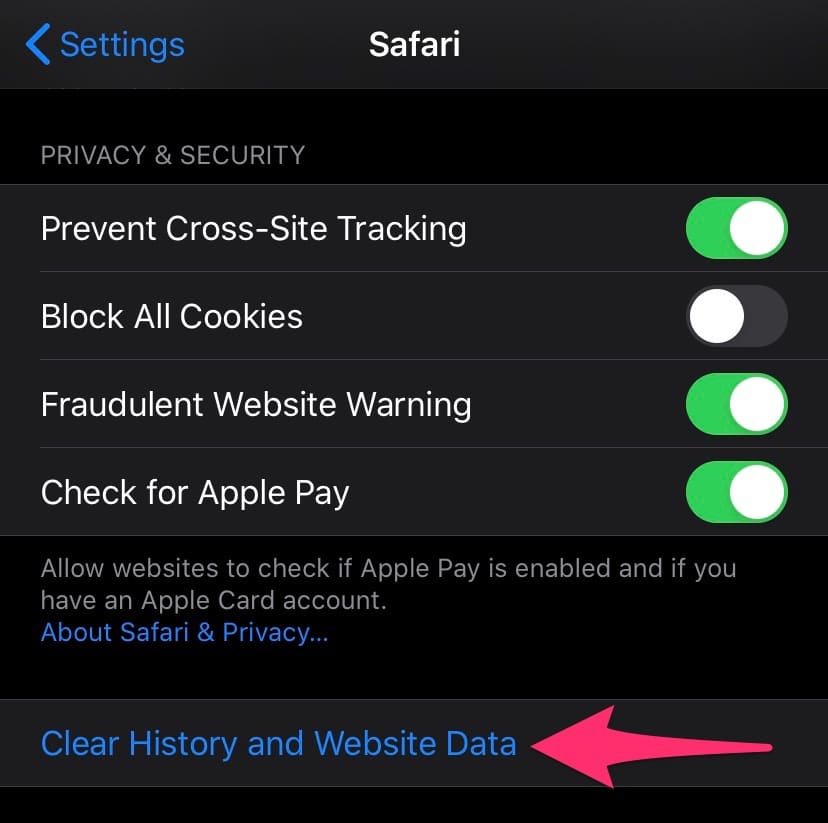The image displays the "Safari" settings on an iPhone, characterized by a sleek black background. At the top, a banner is labeled "Safari," with the word "Settings" in blue on the left, accompanied by an arrow pointing left to navigate back in the settings menu.

Underneath, the heading "Privacy & Security" is prominently displayed, followed by a set of four toggle options:

1. **Prevent Cross-Site Tracking**: This option is turned on, with the switch showing green.
2. **Block All Cookies**: This option is turned off, with the switch showing black.
3. **Fraudulent Website Warning**: This option is turned on, with the switch showing green.
4. **Check for Apple Pay**: This option is turned on, with the switch showing green.

Below the Apple Pay setting, there is a note in light white text: "Allow websites to check if Apple Pay is enabled and if you have an Apple Card account."

Following this, a blue link labeled "About Safari & Privacy" offers additional information. 

At the bottom, a large button appears in a lighter shade of black, with the words "Clear History and Website Data" in blue. To the right of this button, a conspicuous red arrow points towards it, suggesting an action to clear browsing history and data.

The overall aesthetic is uniform with a black-themed background, giving it a polished, modern look.